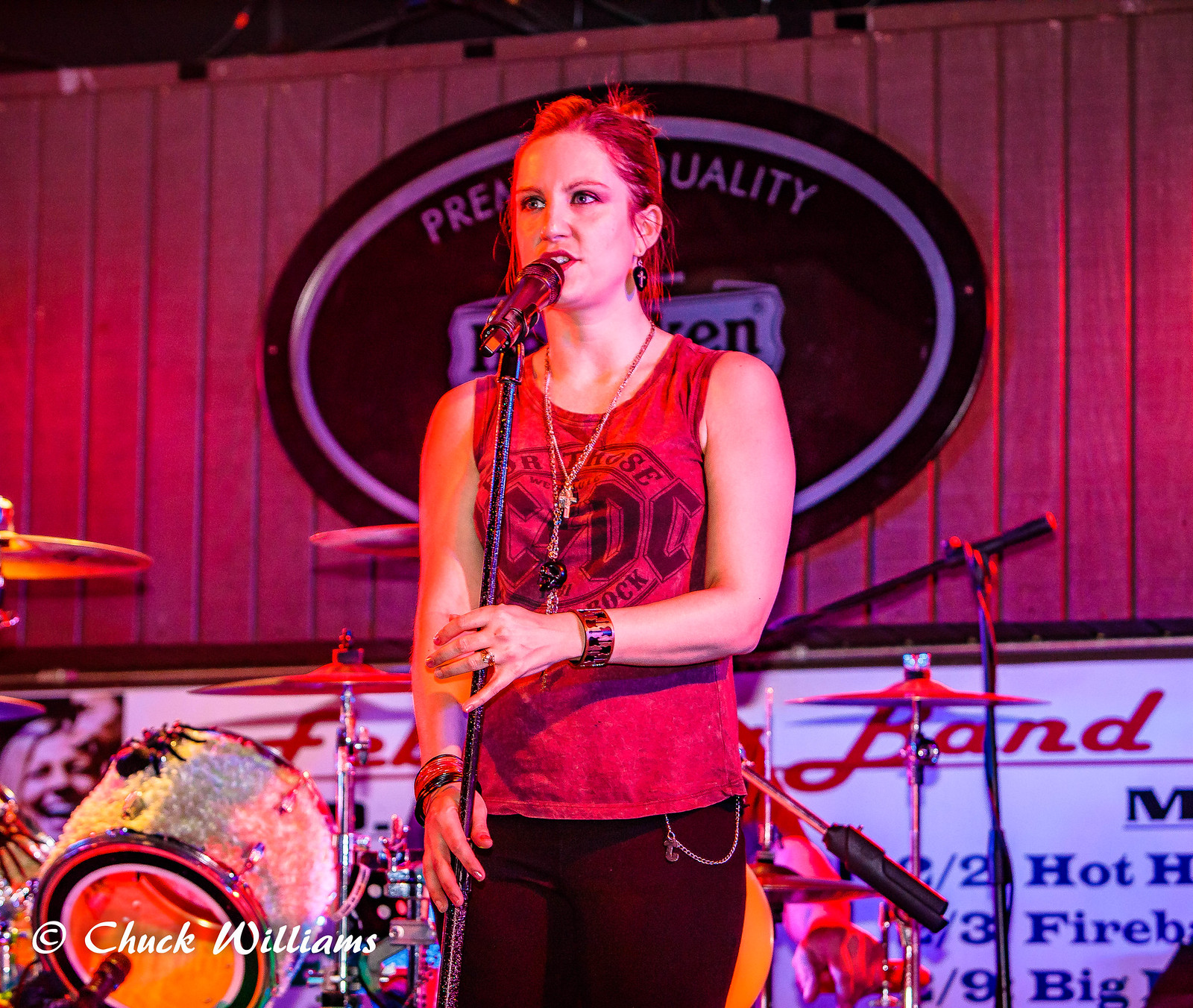The image captures a vibrant scene at a concert or event, possibly a fundraiser, with a young woman at its center. She is standing on a stage, speaking or singing into a black microphone on a stand, her gaze slightly to the left. The woman, who has medium-length blonde or light brown hair styled back, is sporting a red sleeveless tank top emblazoned with "ACDC" in bold black letters. Her ensemble includes black pants adorned with a chain, dangle earrings, various necklaces, a red bracelet, and a ring. 

Behind her, a large Heineken sign with "Premium Quality" emblazoned in black font is partially visible, set against a wooden paneling background. The lower portion of the wall is white, featuring colorful words, including "band" in red on the right side. A champagne-yellow drum set with silver cymbals sits directly behind her, adding to the musical atmosphere of the scene. The entire setting is bathed in numerous colors—black, white, gray, red, pink, blue, yellow, champagne, and silver—enhanced by the stage lighting that highlights her presence.